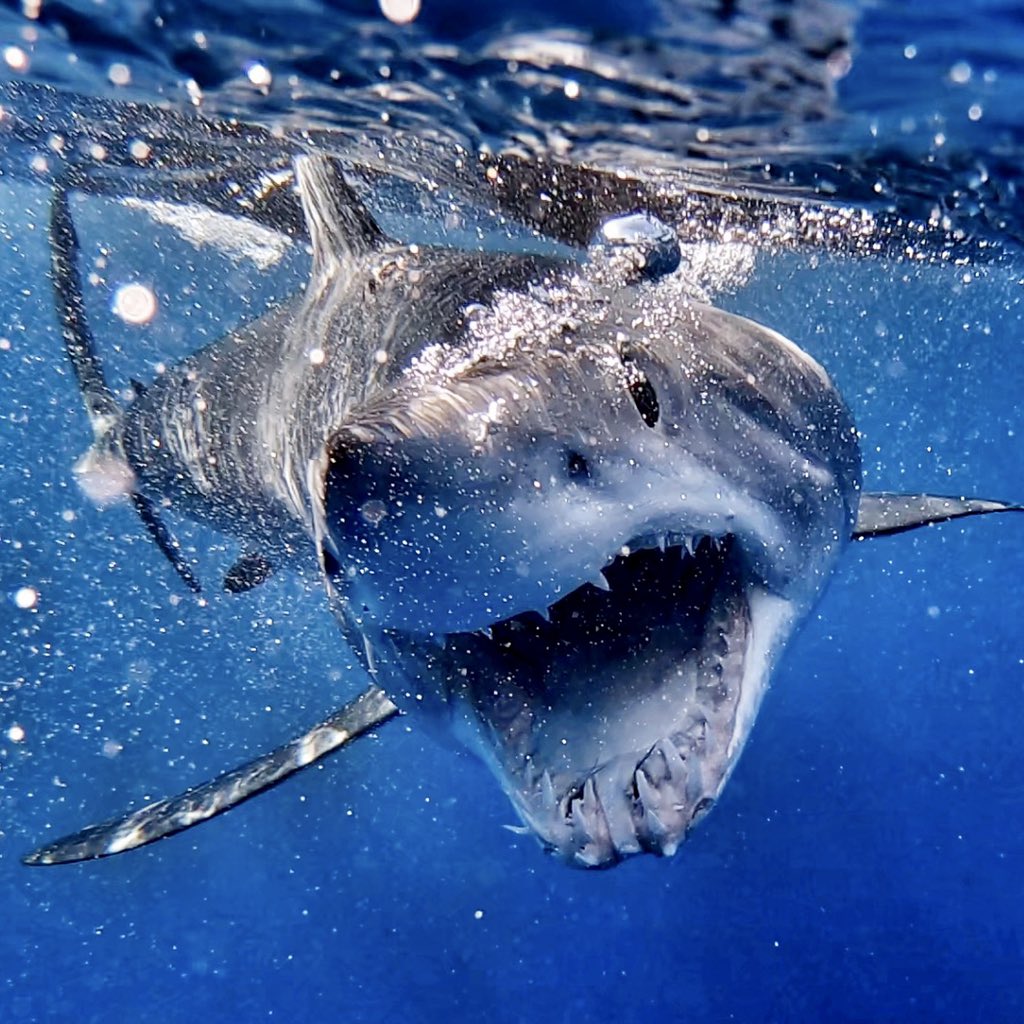This image captures a light gray and white shark swimming directly towards the camera through clear, blue ocean water. The shark's mouth is wide open, showcasing its sharp teeth and even some of the interior of its mouth. One of its eyes and both nostrils are visible, giving the impression that it's intently focused on its path. The photograph highlights the dynamic motion of the scene, with bubbles surrounding the shark, likely stirred up by its swift movement. Its tail fin and dorsal fin break the water's surface, causing waves and ripples. Two smaller fins are seen beneath its body, contributing to the sense of depth and realism in the picture. The water is predominantly blue and appears bright and alive with the shark being the sole subject in the scene. The overall feeling is one of vibrant motion and raw natural power.